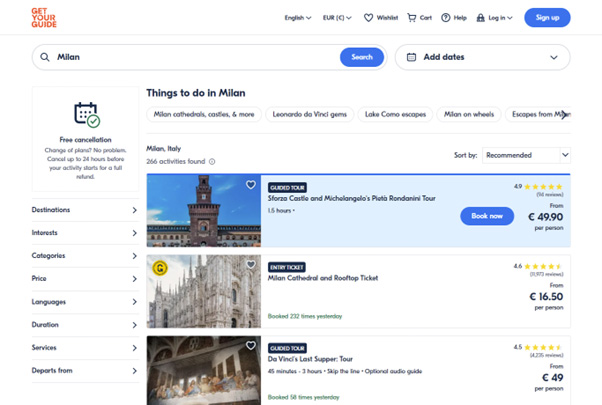The image showcases a user interface from a travel-focused website or application, likely a hotel or tour booking platform. The layout is visually organized, starting with the top left where a prominent "Get Your Guide" logo in orange is situated. Adjacent to it, the search functionality is displayed, with the user having typed in "Milan." To the right of the search box, options for selecting dates are available, likely utilizing a dropdown calendar interface.

Further along the top bar, language and currency options can be customized, with English and Euro set as defaults respectively. Iconic cart and login functions are present, allowing users to manage their bookings and account. A "Sign Up Now" button is prominently placed for new user registrations.

The main content area features a section titled "Things to Do in Milan," listing various activities and attractions. Three notable churches are highlighted, each with distinct pricing ranging from approximately 50 Euro to 16.5 Euro. Customer ratings are visible, represented by a star system on a scale of one to five.

On the left sidebar, multiple filtering options are available, enabling users to refine their search based on destinations, interests, categories, and price ranges. This comprehensive layout ensures a user-friendly experience for individuals planning activities and tours in Milan.